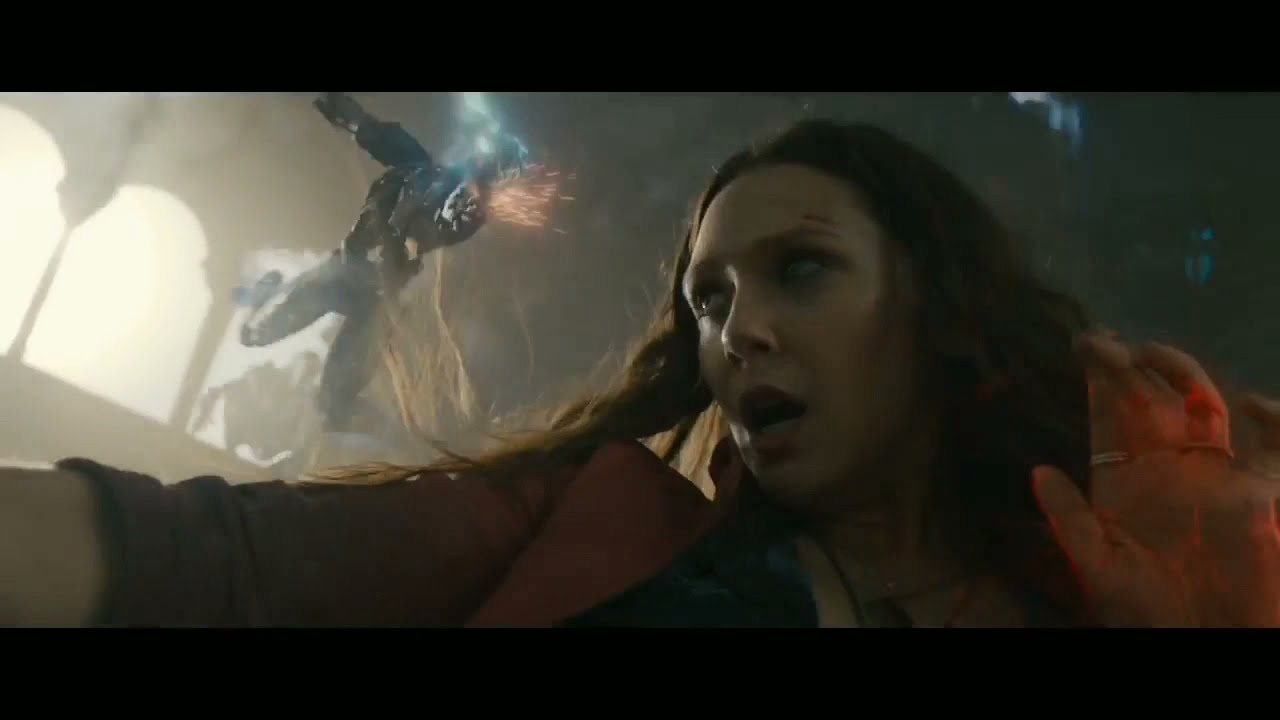The image depicts a dark and dramatic scene possibly from an action movie or a video game, featuring a woman with long wavy reddish-brown hair, blood on her forehead, and cuts above her eye. She appears frightened, holding her hand up with rings on her forefinger and middle finger while her hand is covered in blood. She's standing in the center of a large, dimly lit building or cathedral with external light filtering through the windows on the left side. In the background, there is a menacing figure or creature, possibly wearing a helmet, seemingly hovering or leaping in the air with fiery sparks or flames emanating from what might be a weapon they are holding. The composition suggests the woman is in imminent danger, creating a tense and suspenseful atmosphere.